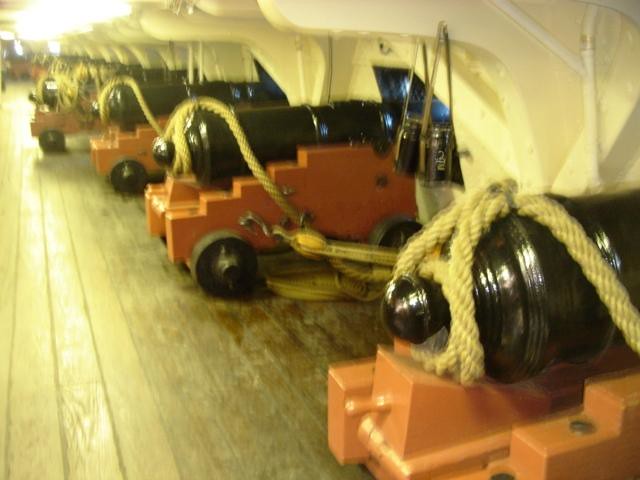The image is a somewhat blurred color photograph depicting the interior of a ship, possibly a museum ship open for tours. It shows several cannons mounted on replica carts, lined up along a wooden floor. Each cart, painted orange or red, features a unique stepped or ziggurat-like design on the sides, and is equipped with wooden wheels secured with cotter pins. The carts hold black cannons, with their barrels protruding through square windows or openings in the white enclosure, mimicking the hull of a ship. Thick ropes, reminiscent of those used to secure ships at port, are wrapped around the butt ends of the cannons and are interconnected, likely to prevent movement when the ship is in motion. Shiny metal components are visible on at least one of the carts, and cargo strapping secures the cannons to the walls. The setting includes a low white ceiling with bright lighting and wooden plank flooring, suggesting an indoor, carefully staged display area.